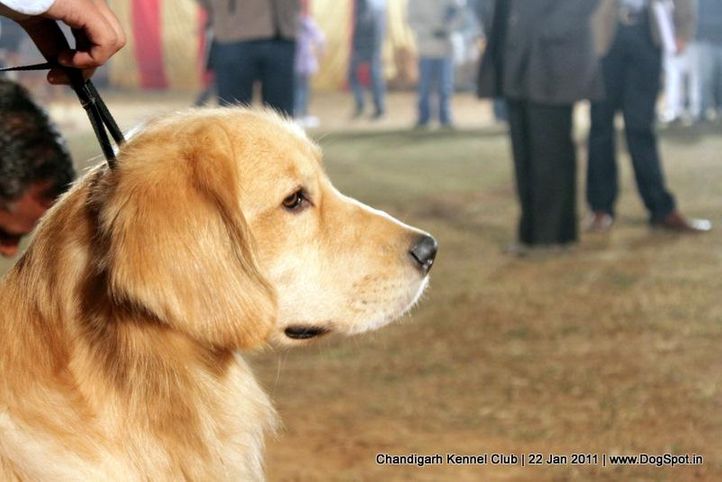The image showcases a golden retriever in a detailed profile portrait, occupying the lower left corner. The dog's tan and slightly white coat stands out as it intently gazes to the right, with a person's hand holding a leash visible beside it. The background is a blurred mix of human legs dressed in black pants, jeans, and brown shoes, suggesting a crowd. The scene appears to be an outdoor event, potentially on worn grassy ground. At the bottom of the image are the words "Chandigarth Kennel Club, 22 January 2011, www.dogspot.in," indicating the photo was taken during a kennel club event on this date.